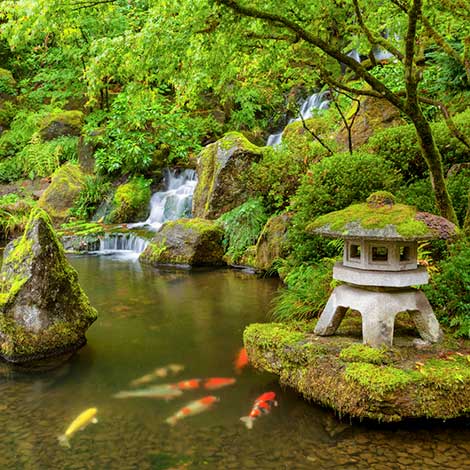The image portrays a tranquil koi pond set within a meticulously manicured, verdant environment reminiscent of a Japanese garden. The pond is teeming with colorful koi fish, including orange, yellow, and striped varieties, prominently visible near the water’s surface. The serene setting features a distinctive stone lantern sculpture with a moss-covered octagonal top, positioned on a rock among other moss-laden stones in the lower right corner. Surrounding the pond, the lush greenery includes abundant trees and bushes, creating a peaceful atmosphere accentuated by the presence of cascading waterfalls in the distance. The photo captures a harmonious blend of nature and carefully designed landscaping, making it an ideal spot for meditation and relaxation.